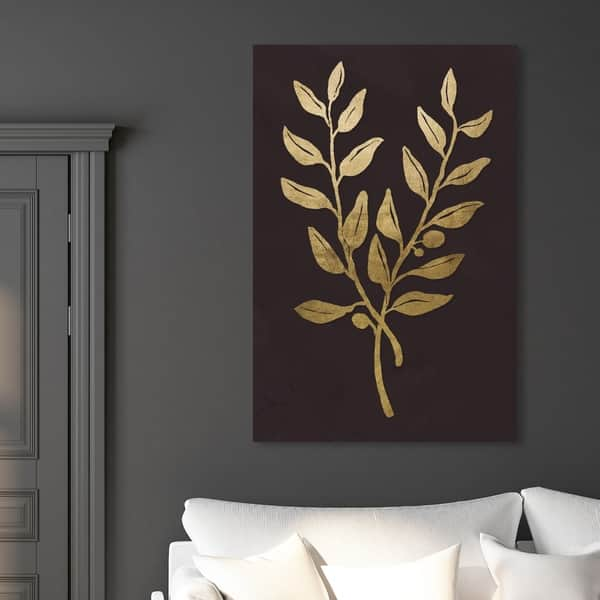The photograph captures a tastefully minimalistic living room painted in deep gray, including the door and its molding which are color washed in the same dark shade. Dominating the foreground is a white couch adorned with large white cushions and a few smaller white throw pillows. Above the couch hangs a large and striking piece of art: a canvas with a dark, maroon background featuring an elegant design of two gold-leafed branches that intersect each other. The simplicity and stark contrast of the artwork against the muted, monochromatic tones of the room create a visually captivating scene.